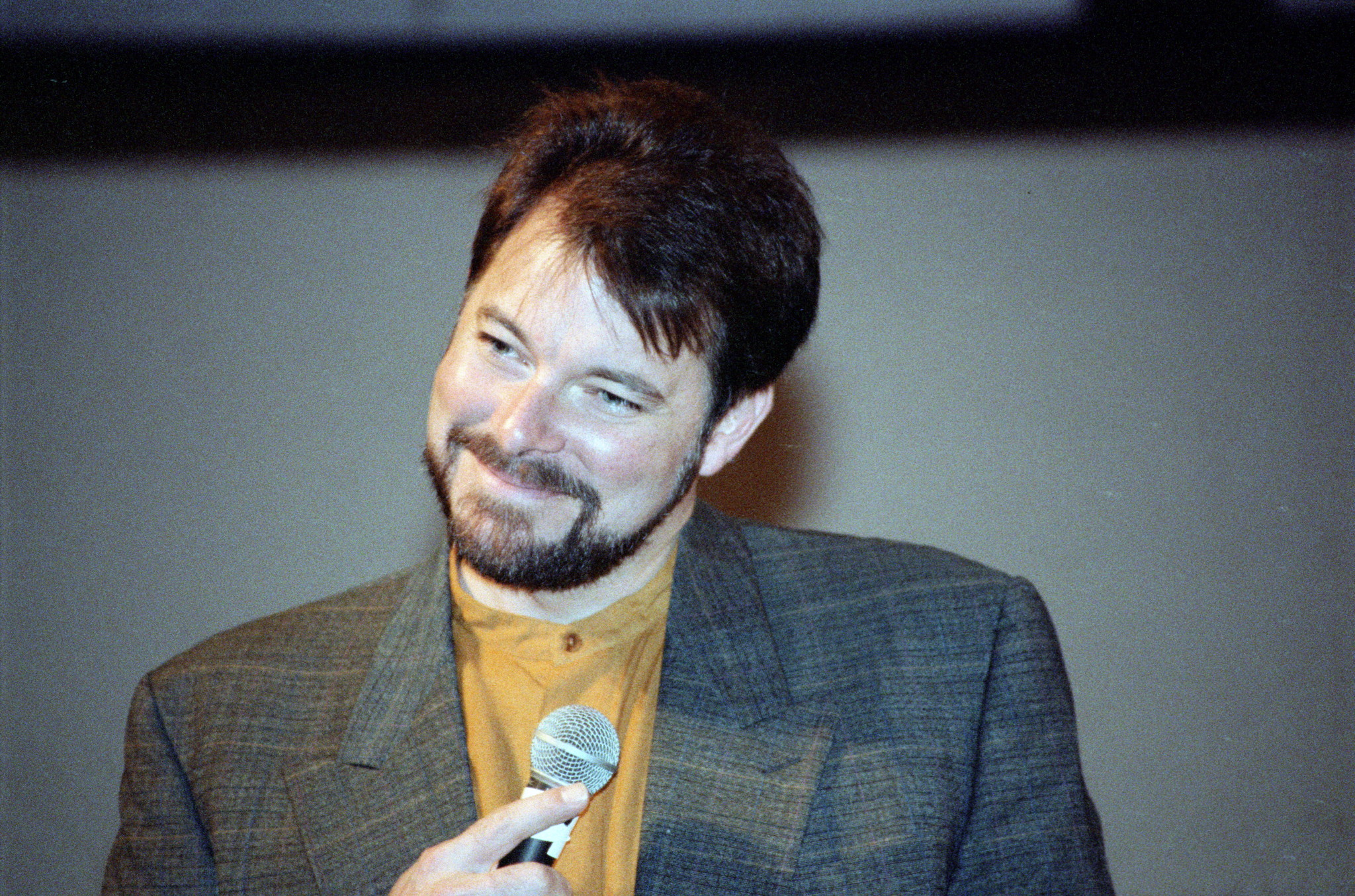In the image, a man with short, slightly poofy black hair and a pencil goatee is seen holding a silver, rounded microphone in his right hand. He is slightly smiling, with his head tilted about 70 degrees to the left, giving off a warm and approachable demeanor. His face features round, slightly rosy cheeks and squinty eyes due to his smile. The man is dressed in a heathered gray suit jacket over a mustard yellow dress shirt with a visible brown button near his neck. The background of the image is predominantly gray, with a black bar running along the upper portion, possibly adding a shadow effect. The wall behind him also reflects a hint of his shadow.